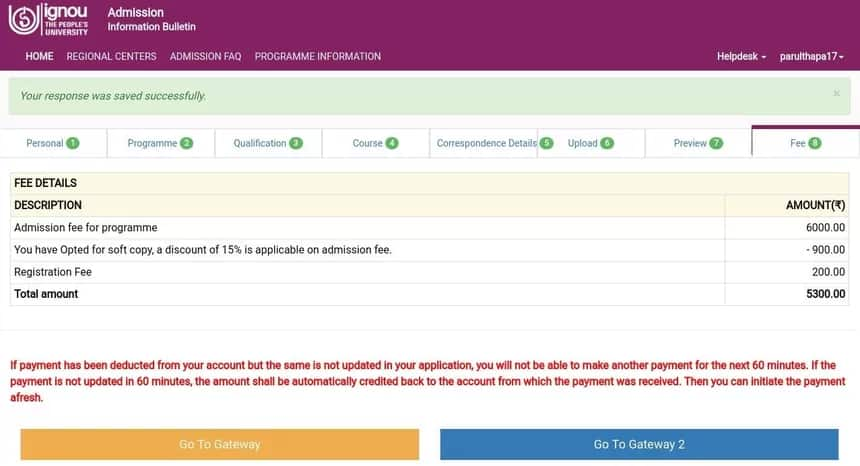This is a detailed caption for the given image:

---

The photograph displays a web page from the Indira Gandhi National Open University (IGNOU), known as "The People's University." At the top of the page, there is a prominent purple banner with white text displaying "IGNOU" and "The People's University." Immediately below the banner, there are options such as "Admissions," "Information Bulletin," and a circular logo featuring an 'S' design at its center. 

The web page has several navigation buttons clearly visible, including "Home," "Regional Centers," "Admission Facts," "Program Information," and "Help Desk." The user's account information is shown, with the name "Parul Thapa, 17" noted.

Further details include sections labeled "Personal," "Program Qualification Course," "Correspondence Details," "Upload," "Preview," and "Fee." At the top of the section, a confirmation message states, "Your response was saved successfully."

In the fee details description, the admission fee for the selected program is listed as $6,000. The user has chosen to pay via "SoftPay," which offers a 15% discount, saving them $900. Additionally, a registration fee of $200 is applied, bringing the total amount due to $5,300. A conspicuous blue button labeled "GoToGateway2" is available for proceeding with the payment.

---

This caption provides a comprehensive and refined description of the image, capturing all essential details coherently.